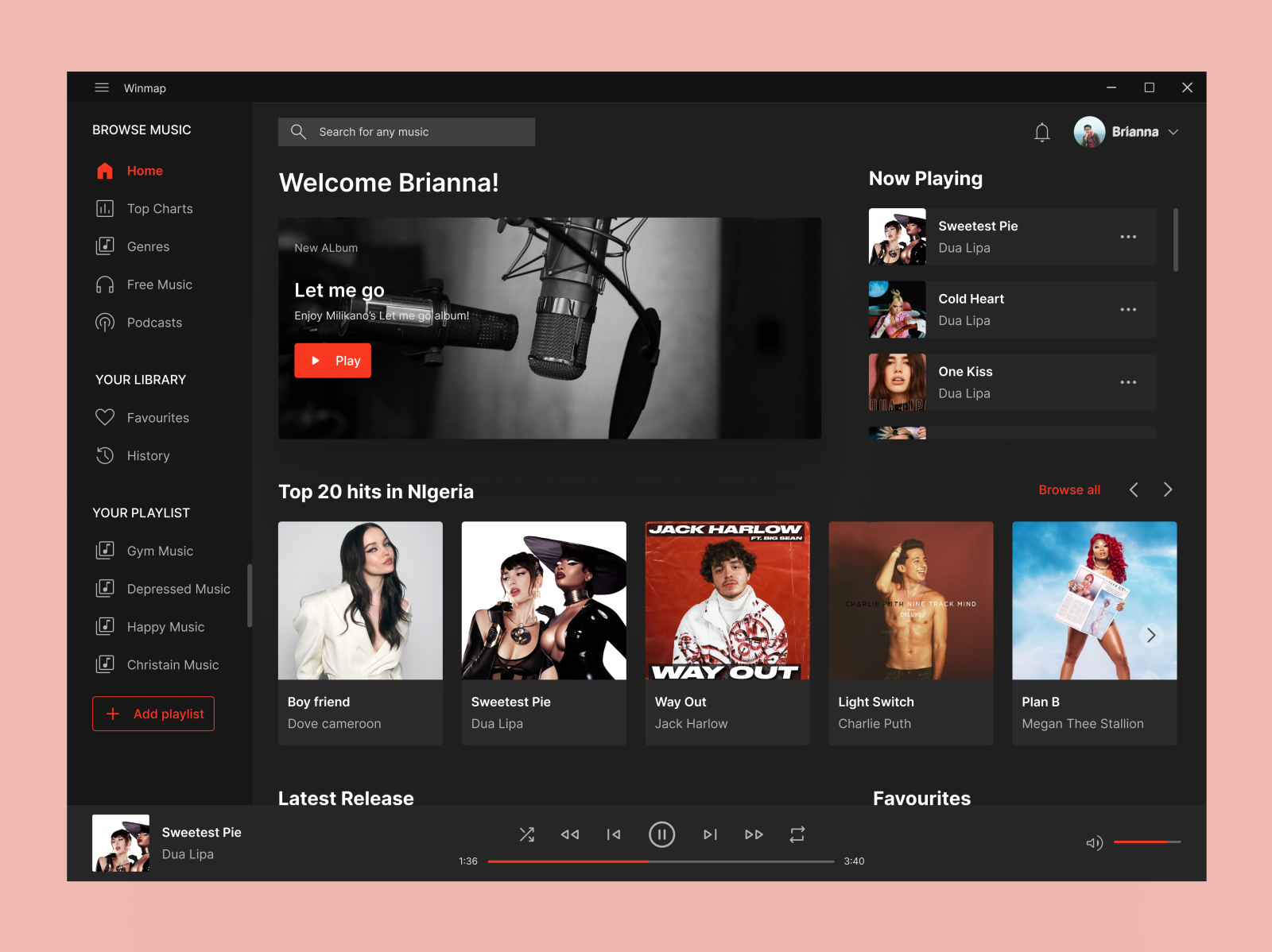This image captures a vibrant interface from a music application, potentially named WinMap or WinApp as indicated by the top left corner of the screen. Below the app name, the clear white font displays "Browse Music," while beneath it a red-font section features a home logo. The main navigation options are prominently listed: "Top Charts," "Genres," "Free Music," and "Podcasts," each accompanied by distinctive icons.

Further down, the interface highlights "Your Library," showcasing options for "Favorites" and "History." This is followed by "Your Playlists," which is populated with various personally curated collections such as "Gym Music," "Depressed Music," "Happy Music," and "Christian Music," along with a red button allowing the user to add new playlists. 

To the right of these sections, the user’s information is displayed, welcoming "Brianna." The central part of the interface spotlights a new album titled "Let Me Go," featuring an image of a pair of microphones and a prominent red play button for immediate listening. Adjacent to this, the "Now Playing" section lists current tracks from Dua Lipa, including "Sweetest Pie," "Cold Heart," and "One Kiss."

Below the main content, a section titled "Top 20 Hits in Nigeria" appears in a dark white font, featuring songs such as "Boyfriend," "Sweetest Pie," "Way Out," "Light Switch," and "Plan B," each accompanied by respective album artwork. At the bottom of the image, the playback controls are visible, including options to play/pause, skip forward or backward, and adjust the volume.